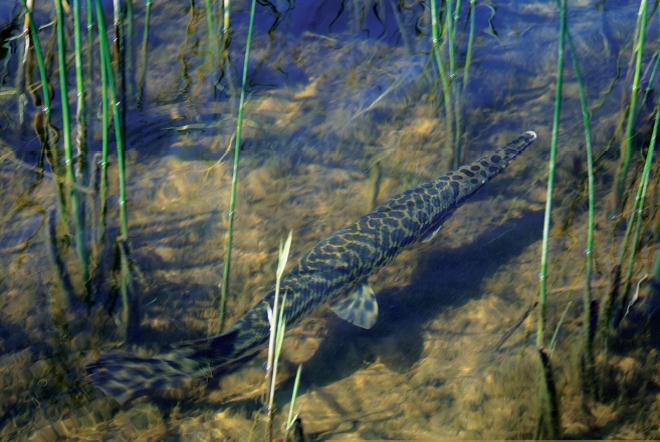In the image, an underwater scene showcases a peculiar, snake-like fish gliding through a shallow body of water. The fish's elongated, slender body is adorned with striking green and black patterns resembling a tiger’s stripes, with some areas featuring cheetah-like black spots on a brownish base. Its body is capped with a long, narrow snout reminiscent of a crocodile's head, and it has a prominent fin near its tail that shares the same vivid design.

The water, a murky green, is clear enough to reveal a yellowed and pale green bottom, interspersed with thin, green, bamboo-like reeds that shoot up towards the surface. These scattered clumps of greenery, found on the left, right, and middle, frame the composition and add a sense of depth. The aquatic plants, much like thick grass or young bamboo shoots, emphasize the shallow nature of this watery habitat, which appears to be only about six inches deep.